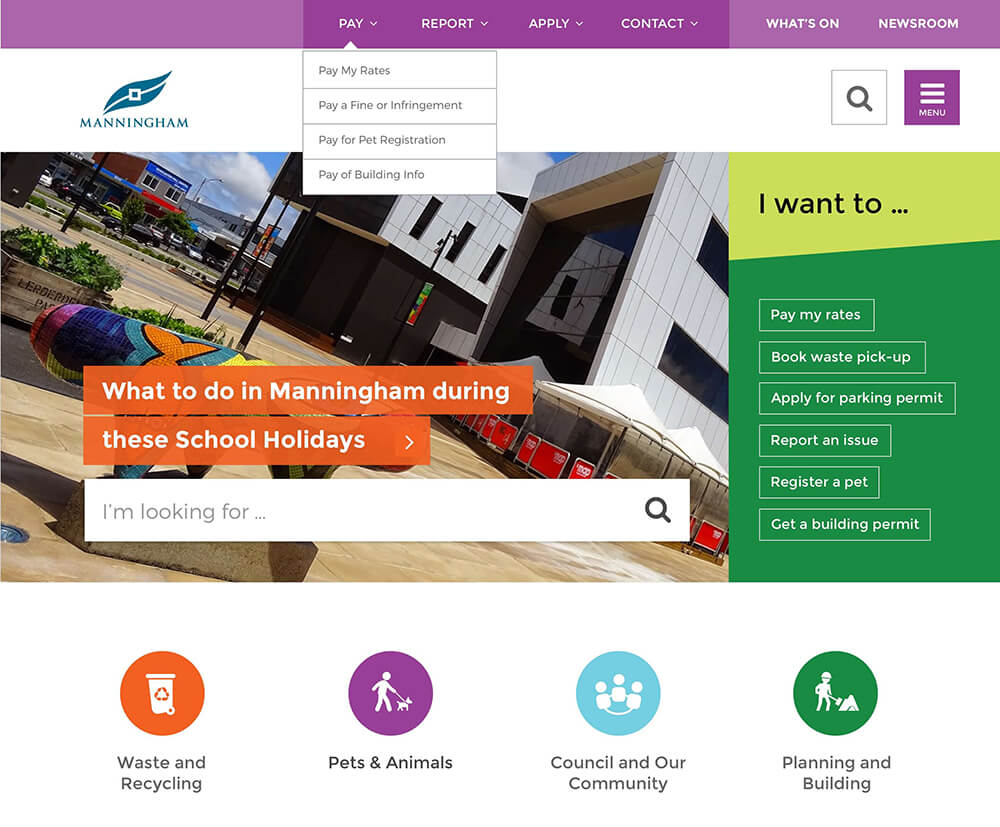The screenshot depicts the homepage of a website named "Manningham." In the top-left corner, it features the Manningham logo and name. The uppermost section of the screen is highlighted by a prominent purple banner extending horizontally, which contains a series of drop-down menus labeled: Pay, Reports, Apply, Contact, What's On, and Newsroom, arranged from the center to the right. 

Below this banner, on a white background where the logo is situated, there are icons for search functionality and a menu option, positioned to the right of the logo. Dominating the left side of the screen is an image of office buildings with two orange stripes and white overlay text that reads, "What to do in Manningham during the school holidays," which serves as the title for a drop-down menu. Beneath this, there is a white editable field inviting users to type in their interests with the prompt, "I'm looking for."

On the right-hand side, a green panel is present, marked at the top with a light green section containing the text "I want to." The lower section of this panel offers multiple actionable options, including: Pay My Rates, Book Waste Pickup, Apply for Parking Permit, Report an Issue, Register a Pet, and Get a Building Permit.

At the very bottom of the main image, four distinct icons are aligned horizontally: one orange icon for Waste and Recycling, a purple icon for Pets and Animals, a light blue icon for Council and Our Community, and a green icon for Planning and Building.